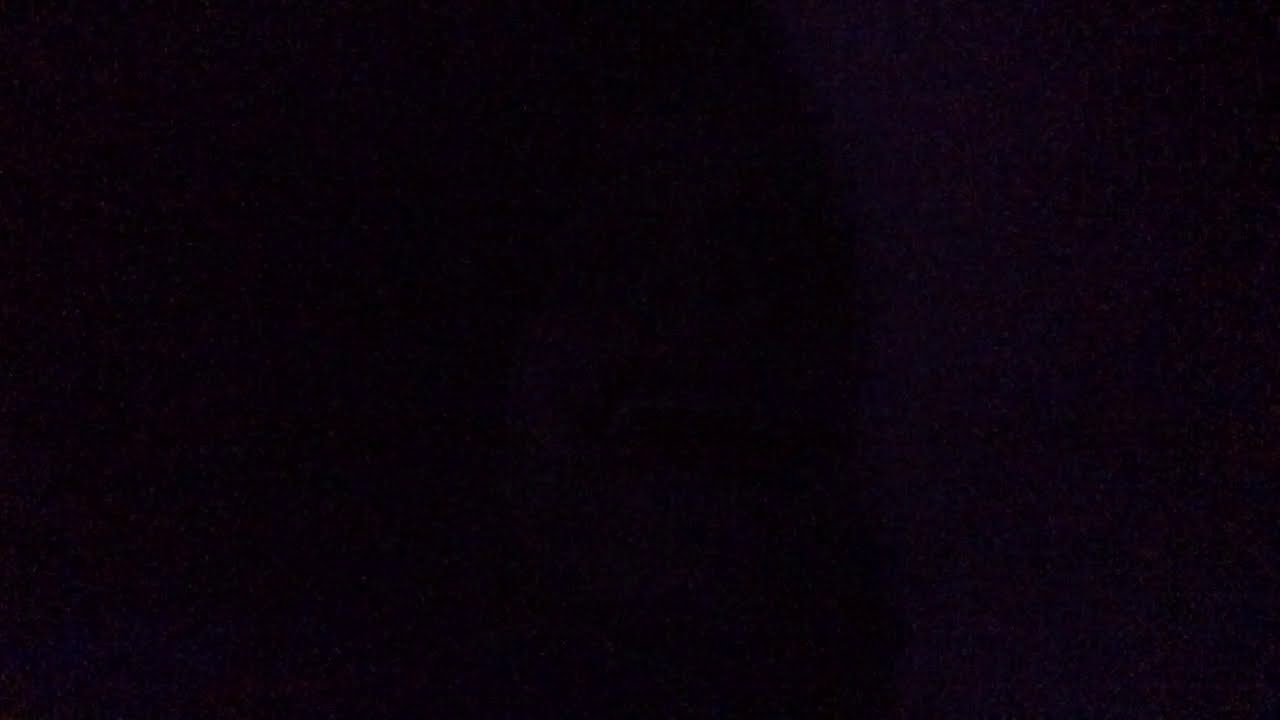The image consists solely of a completely black background, devoid of any objects, text, designs, or patterns. The color black dominates the entire rectangular frame, creating an uninterrupted expanse of darkness from left to right. This could evoke the sensation of being in a pitch-black room or tunnel, the night sky obscured by overcast clouds, or the vast emptiness of space without visible stars or planets. The lack of light and any visual elements in the image only heightens the sense of isolation and absolute void. It's a purely monochromatic scene, emphasizing the depth and all-encompassing nature of darkness.